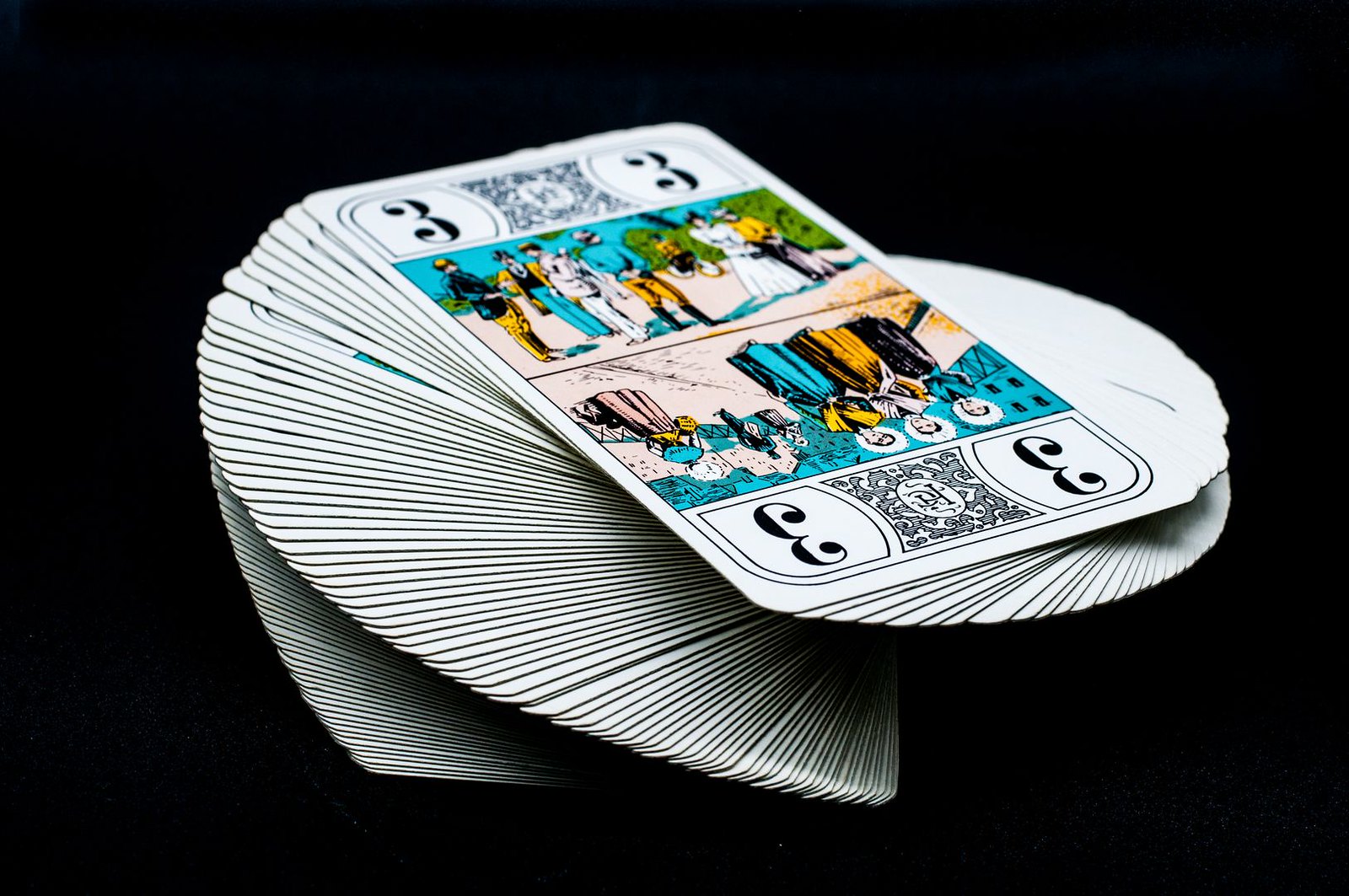This close-up photograph captures a fanned-out deck of tarot cards arranged in a spiral, with a focus on the card at the top. The featured card prominently displays the number three in all four corners. The intricate scene on the card depicts two distinct images: one right side up and one upside down. The right side up image shows a man and a woman standing together, surrounded by various men, some facing the couple while others have their backs turned. The upside down image features three women standing closely together, with a little boy nearby and a man walking away from the scene. The overall background of the photograph is black, and the lighting is dim, creating a mysterious ambiance. The colors on the top card are predominantly blue, gold, and black, with everyone depicted in a combination of these colors along with some white.